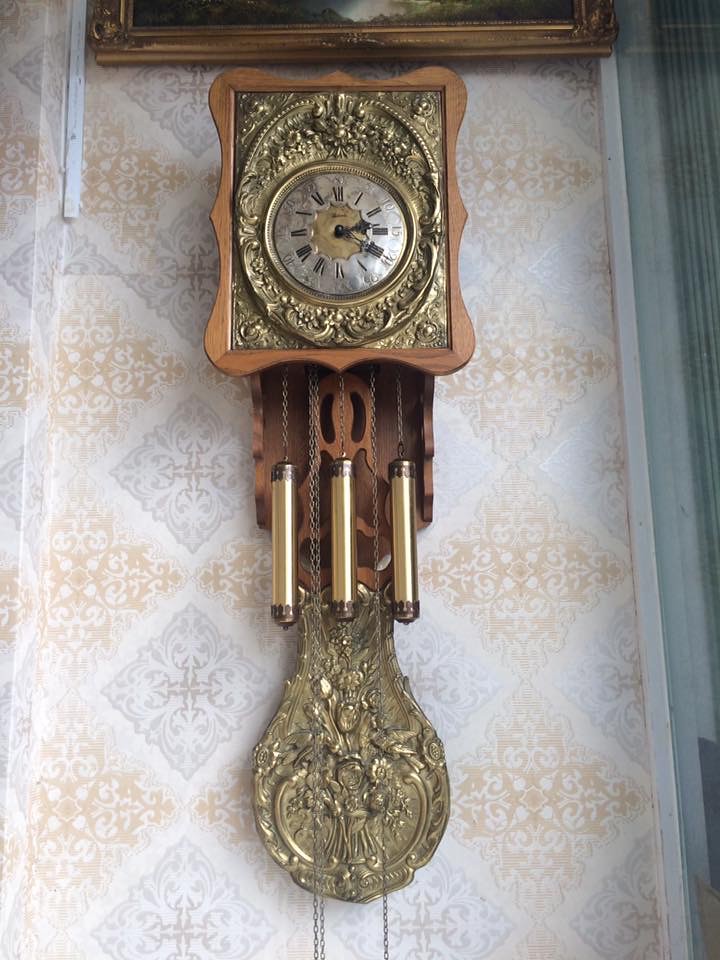This image showcases a rectangular portrait-oriented photograph of an ornate, antique wall clock. The clock prominently features a metallic face with Roman numerals, indicating the time as 2:20. Surrounding the face is an elaborate brass or gold rim with intricate carvings, complemented by a wooden structure that adds to the decorative appeal. The clock's hands are particularly ornate, and the centerpiece of the face includes a multi-pointed star design. Below the face, hanging chimes and a paddle-like structure adorned with gold carvings add to the clock's grandeur. The clock is mounted on a wall covered with a light brown and gray, paisley-like, filigree-patterned wallpaper. Above the clock, a picture frame is partially visible.